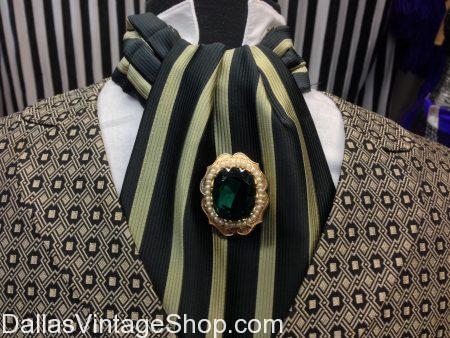This image features a detailed advertisement for DallasVintageShop.com, prominently displayed in white letters at the bottom left of the rectangular, horizontal photo. At the center of the image is a mannequin dressed in a striking men's formal outfit. The ensemble includes a tan and black geometric-patterned jacket, reminiscent of paisley or checkerboard designs incorporating small squares and irregular black circles with white centers. Beneath the jacket, the mannequin sports a high-collared white shirt overlaid by a black and light-green vertically striped ascot, adorned with a dark green jewel centrally set in a gold and possibly diamond-encrusted setting. The background features a black and white striped pattern, adding contrast and emphasizing the vintage aesthetic of the outfit. An additional green pin on the ascot adds a touch of elegance, highlighting the intricate details of this carefully curated ensemble.